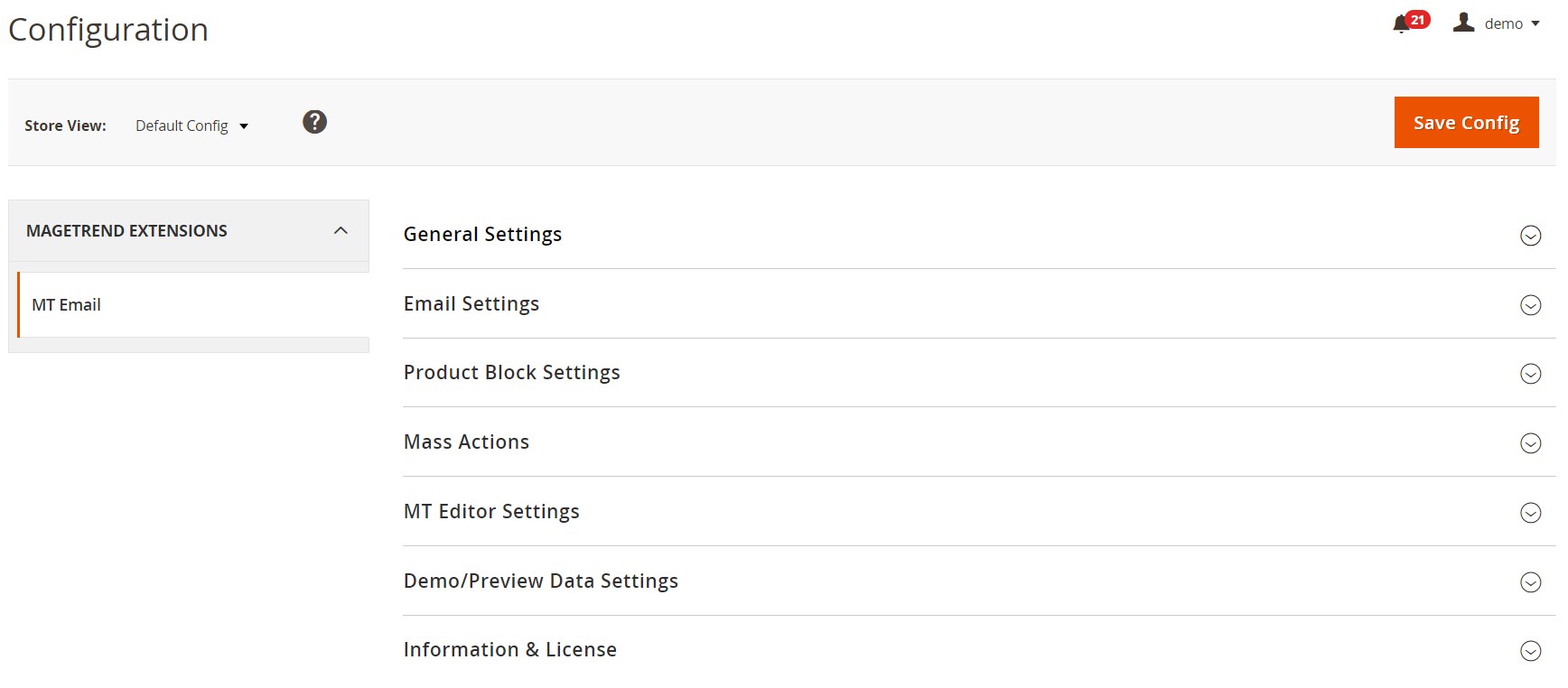The online screen image features a user interface primarily designed for configuration tasks. Positioned at the very top left-hand corner is the label "Configuration." Below it, the section titled "Store Views" is displayed, containing a dropdown box labeled "Default Configuration" indicated by a black downward arrow. Adjacent to this, there is a black circle enclosing a question mark. Directly underneath, there is a tab labeled "Match Trend Extensions," followed by an upward-pointing arrow.

To the side, a submenu lists various settings options, including General Settings, Email Settings, Product Block Settings, Mass Actions, Empty Editor Settings, Demo/Preview Date Settings, and Information and License. 

On the upper right-hand side of the screen, a notification bell icon with a red circle displaying the number 21 is present, indicating new alerts. Next to the bell, there is a profile icon shadowed, labeled "Demo" with a black dropdown arrow beside it. Beneath this, there is an orange banner labeled "Save Config."

The background is plain white, lacking in diverse colors, signifying a back-end system interface. This interface serves as an area where users can make changes or configure various elements within the system.